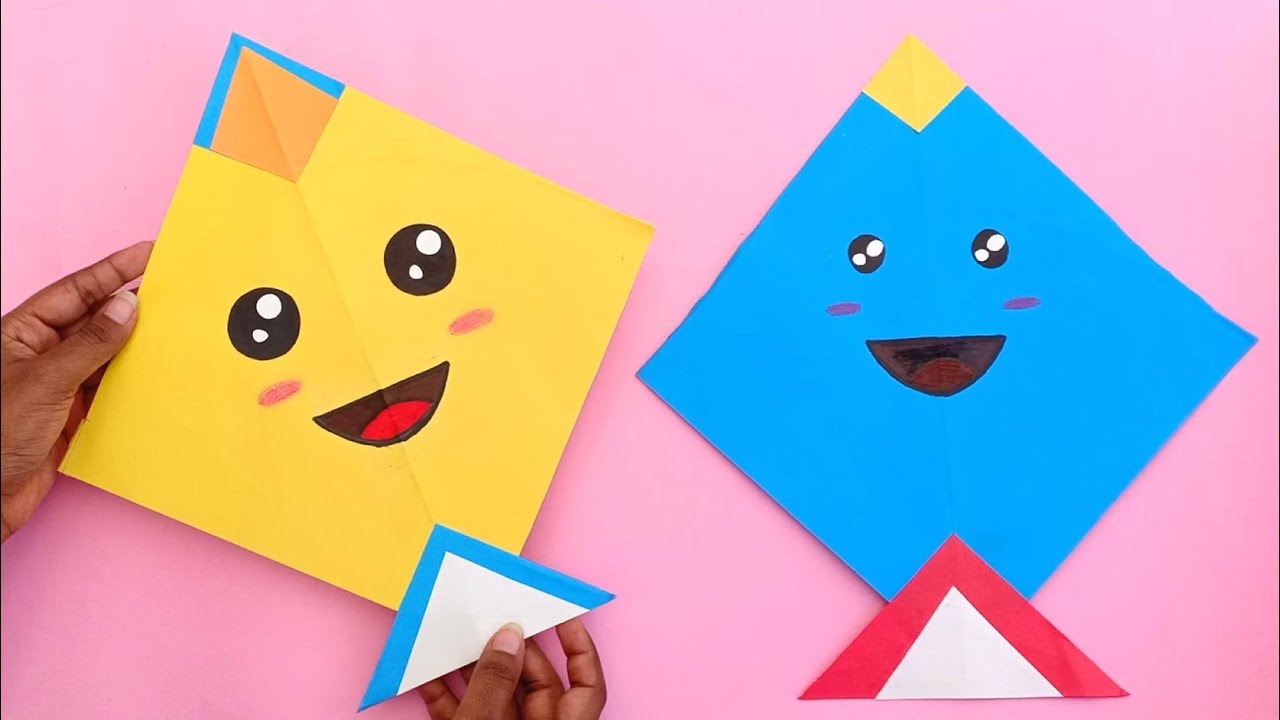The photograph features a tabletop with a light pink covering, showcasing two pieces of kindergarten-level DIY paper crafts positioned as diamonds. The left diamond is yellow and held by the hands of an African American woman, identifiable by her long fingernails. This yellow diamond sports a face with large eyes, each containing white spots, and a smiling mouth. Additional details include a beige diamond edged in blue at the top and a white triangle edged in blue at the bottom.

The right diamond is blue, also displaying a happy face similar in style but with smaller eyes. It features a yellow diamond at the top and a white triangle with red edges at the bottom, likely representing a neck. The artistic effort and the playful arrangement of the colored paper pieces highlight a whimsical and creative approach to crafting.